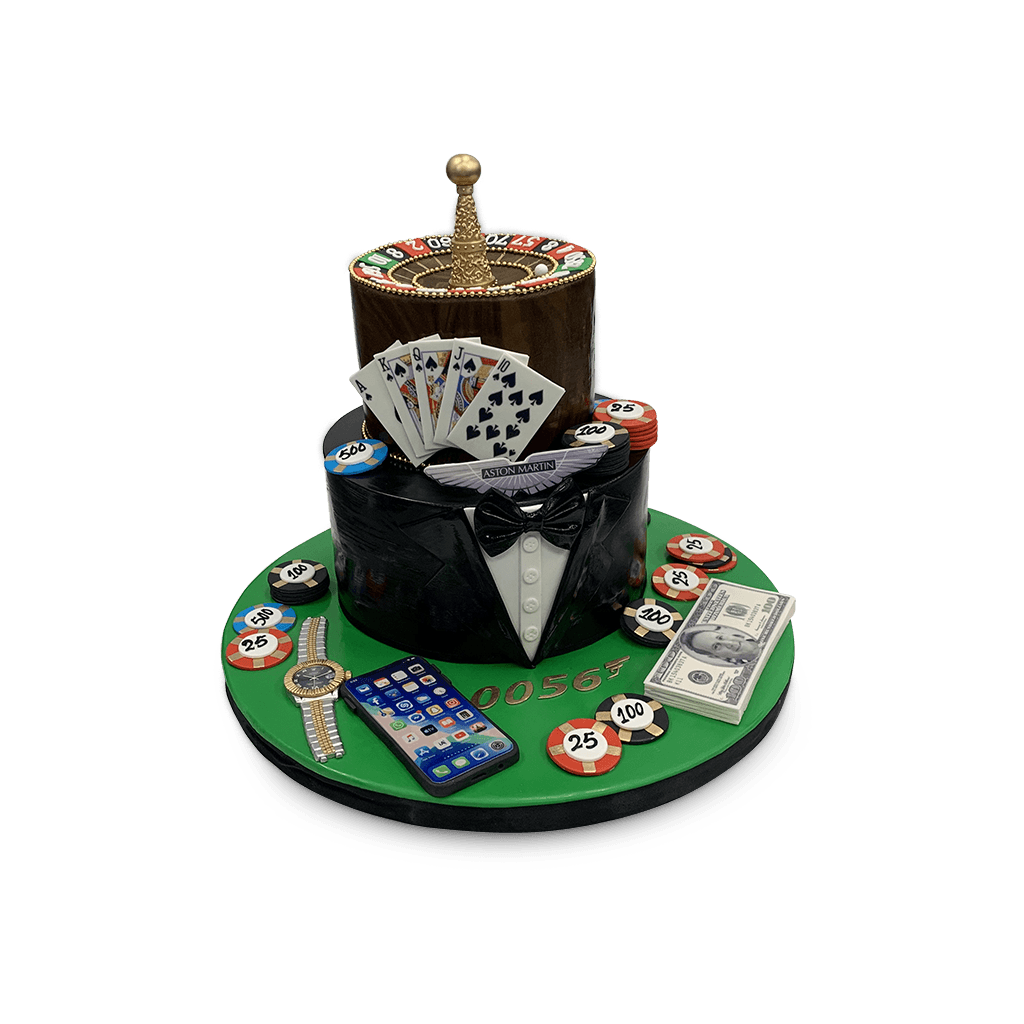The image is a professionally done color photograph, in a square format, depicting a meticulously crafted poker-themed desktop organizer. The subject floats against a seamless white background, emphasizing its detailed composition. At the base, a flat, green circular platform trimmed in black showcases an array of personal items. On the left side rests an open cell phone displaying its icons, paired with a sophisticated Rolex watch. To the right are stacks of poker chips in various denominations, including red $25 chips, black $100 chips, and a blue $500 chip, alongside a pile of currency. 

At the center of this platform stands a taller round structure fashioned to resemble a tuxedo with black lapels, a plastic bow tie, and white shirt buttons. Atop this tuxedo-shaped tower, a fanned hand of cards (10 through Ace of Spades) is displayed. The apex of the structure is crowned with a smaller black circular base bearing a luxurious roulette wheel. The roulette wheel, bordered by pearls and featuring a gold Christmas tree-shaped pyramid at its center with a small gold ball, adds an elegant touch to the composition. A winged Aston Martin logo is prominently displayed above the bow tie on the tuxedo. The overall style of the image is photographic realism, oriented towards product photography, capturing the intricate details and luxurious elements of the poker-themed arrangement.